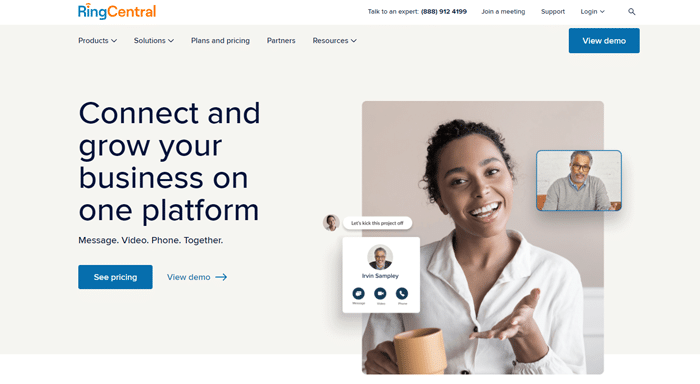In the top-right corner of the image, the text "RingCentral" is prominently displayed, with "Ring" in blue and "Central" in orange. To the right of this, the text reads "Talk to an expert, 888-912-4199," followed by options to "Join a meeting," "Support," and "Log in." A magnifying glass icon for search is also visible. Below these options, a navigation bar includes links labeled "Products," "Solutions," "Plans and Pricing," "Partners," "Resources," "View Demo." 

The main section of the image features a tagline: "Connect and grow your business on one platform—message, video, phone, together." Beneath this, buttons for "See Pricing" and "View Demo" are displayed, alongside an arrow pointing to the right.

The central photograph showcases a young dark-skinned woman with short dark hair, smiling directly at the camera. She is dressed in a white collared shirt and holds an orange coffee mug in her right hand, while her left hand is raised.

To the right of this main image, there is a smaller photograph of an older dark-skinned man wearing black-framed glasses and a gray sweater. To the left, a circular icon displays the same woman from the main image above the text "Let's kick this project off."

Below this circular icon, a white square contains a smaller photograph of the same man. Beneath his photo, the text reads "Ervin Sampley."